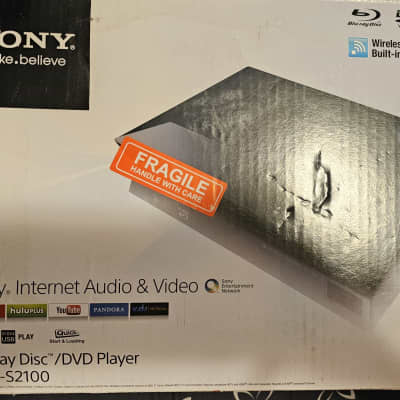This image features a detailed look at a portion of the Sony Blu-ray Disc DVD Player, specifically model S2100. The square photograph prominently displays the cropped Sony logo in the upper left corner, showing the last three letters 'ny' in white on a black background. In the upper right corner, a partially visible Bluetooth wireless symbol—a 'B' combined with a crescent—can also be seen, similarly cropped.

Centrally aligned towards the right is a photograph depicting an object that might either be the player itself with a noticeable dent in its packaging or something resembling a wallet placed inside a cardboard box. Adding to this scenario is a red "Fragile - Handle with Care" sticker positioned over the object, near the left side of the dent in the box.

In the lower left quadrant, the image contains text partly revealing the features of the device, mentioning "internet, audio, and video." Below this, small rectangular icons representing various streaming services, such as YouTube, Pandora, and Hulu, are displayed—indicating the player’s capabilities to offer diversified multimedia content.